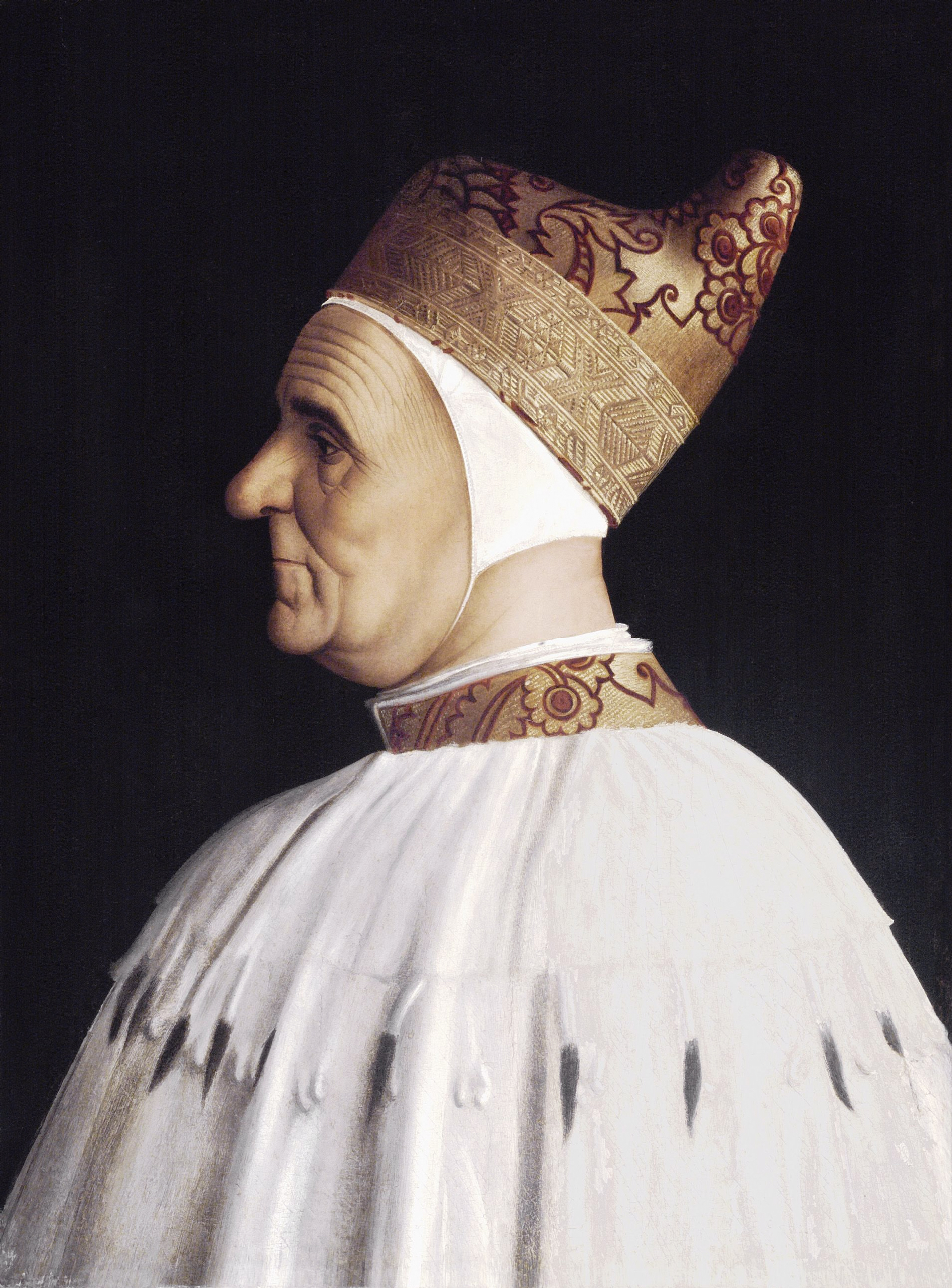The image is a detailed color portrait titled "Doge Giovanni Mocenigo" by Gentile Bellini, created circa 1478, and showcases Renaissance Realism. It features an elderly male member of the clergy, depicted in a serene side profile facing to the left, with a prominent, long nose and a wrinkled brow, emphasizing his stern and distinguished demeanor. He is attired in a white cassock accented with delicate feather trim around the neckline and brown tassels. His headgear is a notable gold and burgundy silk cap adorned with scroll embroidery, which extends to a pointed top at the back, complemented by a wide band of beige embroidery around his forehead. This elaborate hat fits over his head and is secured under his chin with a white cloth, which also covers his ears. The detailed depiction captures both the intricate fabric textures and the dignified air befitting a clergyman of the 15th or 16th century.